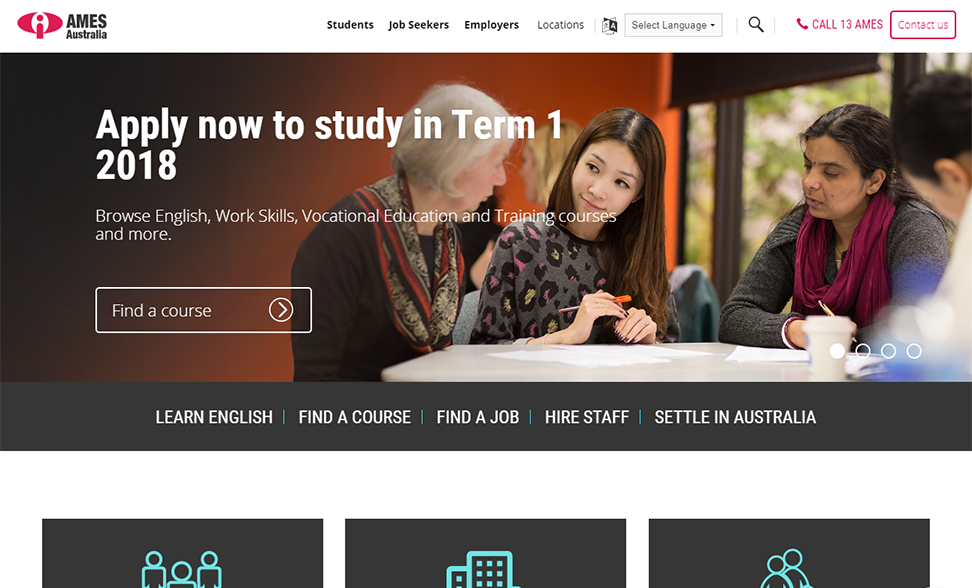**Caption for the Image:**

The online advertisement has a clean and structured design divided into several sections, starting with a top banner which is set against a white background. On the leftmost side of the banner, there's a distinctive red circle with an eye symbol centered within it. Next to this emblem, "Ames Australia" is prominently displayed in black font. Moving rightward, there are text snippets in varying shades, with "students," "job seekers," and "employers" marked in black, while "locations" is noted in gray font. 

Adjacent to this text area is a gray and white square featuring a drop-down menu labeled "Select Language." Right beside it, there's an icon of a magnifying glass symbolizing the search function. A notable feature here is a vibrant pink square displaying a phone icon with the text "Call 13 Ames," all in pink, alongside another pink box with the message "Contact Us."

Directly below the banner, another larger image catches the eye. It starts with a black background that gradually transitions into shades of brown, then light brown, encapsulating the setting of a casual, yet informative scene where a couple of women are sitting at a table, engrossed in conversation. Superimposed on this background in white font is the call to action: "Apply now to study in Term 1, 2018." Below this, the text invites potential candidates to "Browse English, work skills, vocational education and training courses, and more."

Further enhancing the navigation experience, a white box presents itself with the label "Find a course," accompanied by a white circle and right arrow. Positioned beneath this box, a sequential list in white font on a grayish line reads: "Learn English," "Find a course," "Find a job," "Hire staff," and "Settle in Australia," each separated by a blue line.

At the bottom, three square-shaped images are seen: the first features a probable depiction of people in teal blue, the second square illustrates a series of buildings with visible windows, and the third image portrays two individuals.